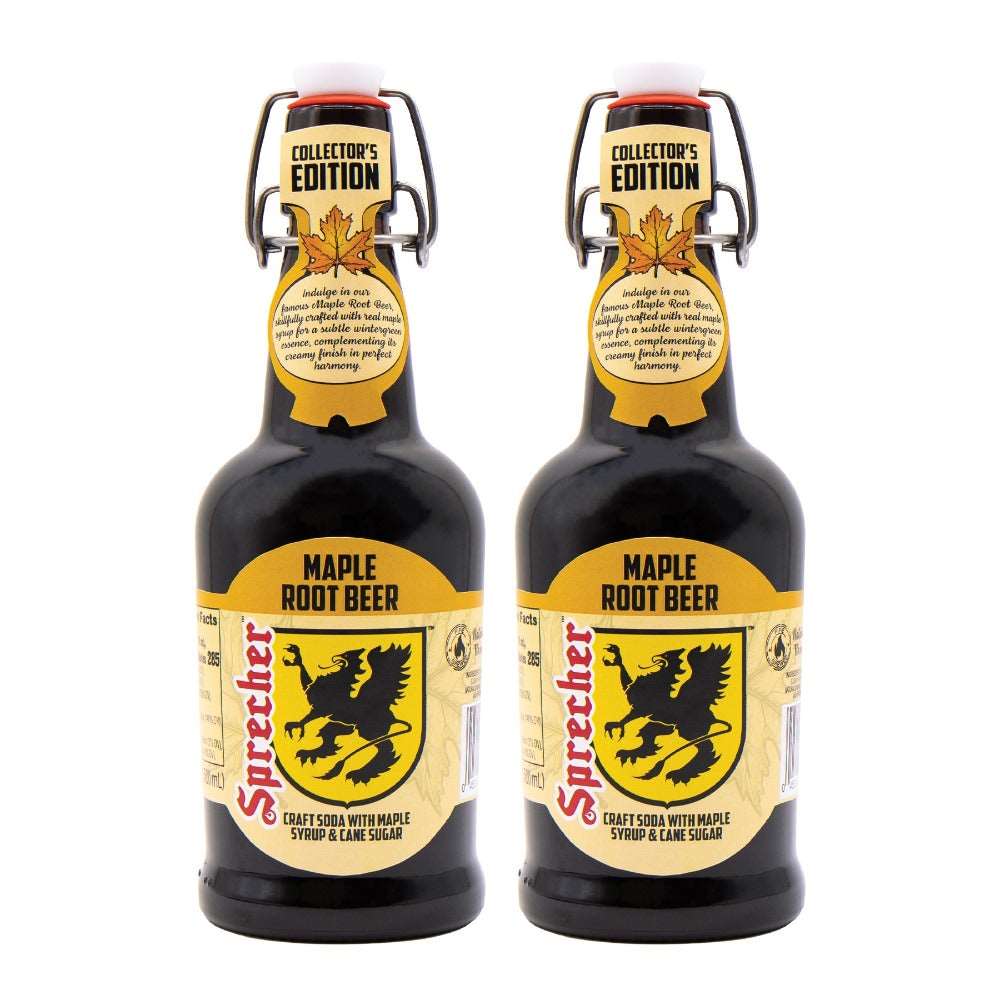The image showcases two glass bottles of maple root beer, positioned side-by-side against a white background, with their fronts facing forward. Each bottle is a Collector's Edition, as indicated by the text on their distinctive red-and-white flip-top lids. The bottles, designed with an old-fashioned pop lock clasp, feature a label that prominently displays a maple leaf below the "Collector's Edition" notice. The bottles themselves are a dark color, likely black, and the labels incorporate a rich palette of orange, yellow, and black tones.

Centrally placed on the front of each bottle is a stylized yellow shield adorned with a black dragon, reminiscent of a heraldic crest. Above this is the brand name, "Sprecher," written diagonally in bold red text. Just beneath the dragon crest and brand name, small black lettering declares the product as "craft soda with maple syrup and cane sugar." The labels also prominently state "maple root beer" in black text set against a yellow background. Overall, the presentation exudes an artisanal, local, and individualistic character, appealing to collectors and connoisseurs of unique craft sodas.